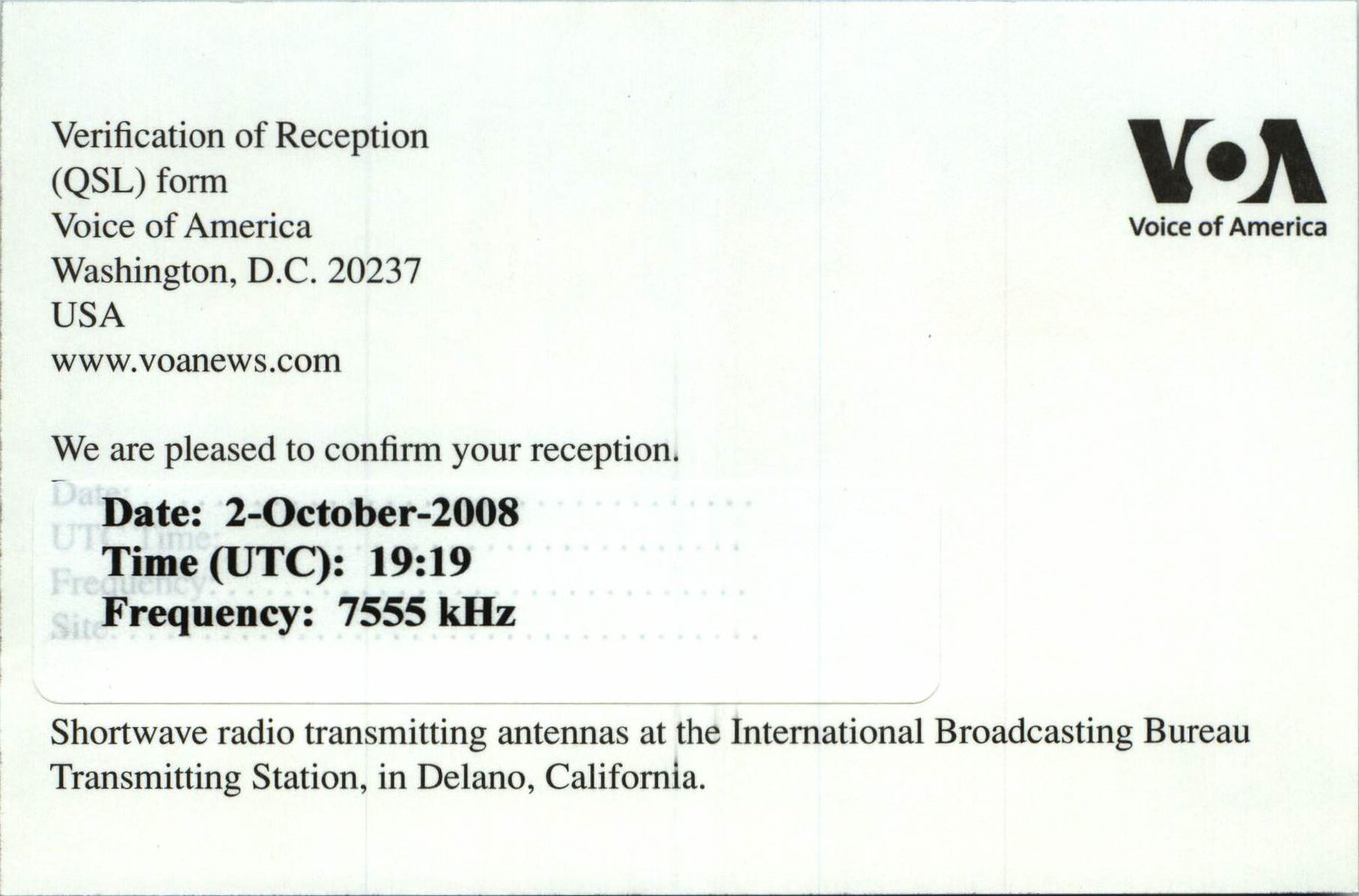The image depicts a landscape-oriented verification of reception postcard from Voice of America (VOA). The postcard features a faint, thin black pinstripe outline around its white background. The top right corner prominently displays the VOA logo: a black "V" and "A" with a white "O" encircled in black. Below the logo, the text "Voice of America" is printed in smaller font. On the top left side, the postcard bears the heading "Verification of Reception (QSL form)," followed by the address "Voice of America, Washington DC, 20237, USA," and the URL "www.VOANews.com." Below this, it states, "We are pleased to confirm your reception," followed by the date, time, and frequency details in bold print: "Date 2-October-2008 Time (UTC): 19:19 Frequency: 7555 KHZ." Further down, there's a descriptive line stating, "Shortwave radio transmitting antennas at the International Broadcasting Bureau transmitting station in Delano, California." The overall style resembles a printed collateral or publication, confirming the successful reception of a radio transmission.